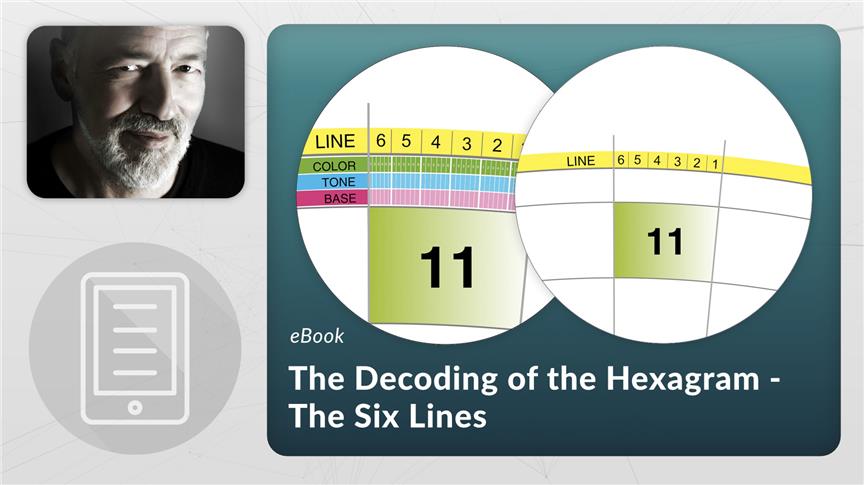The image is a PowerPoint slide or presentation with a predominantly white background. In the top-left corner, there's a photo of an older white man with a white beard and a black shirt, appearing somewhat confused, with a shadow cast over the left side of his face. Below his photo is a simple cartoon depiction of a tablet enclosed within a gray circle.

Most of the image is dominated by a dark green or aqua blue square featuring a Venn diagram with two white circles filled with lines in green, blue, and red, labeled with "line," "color," "tone," and "base." To the left of the circles is the number 11 in black text, mirrored on the right side. Beneath this diagram, the text "e-book" is displayed in white, followed by "the decoding of the hexagram, the six lines" in white text as well, suggesting this is an advertisement for an e-book focused on decoding hexagrams.